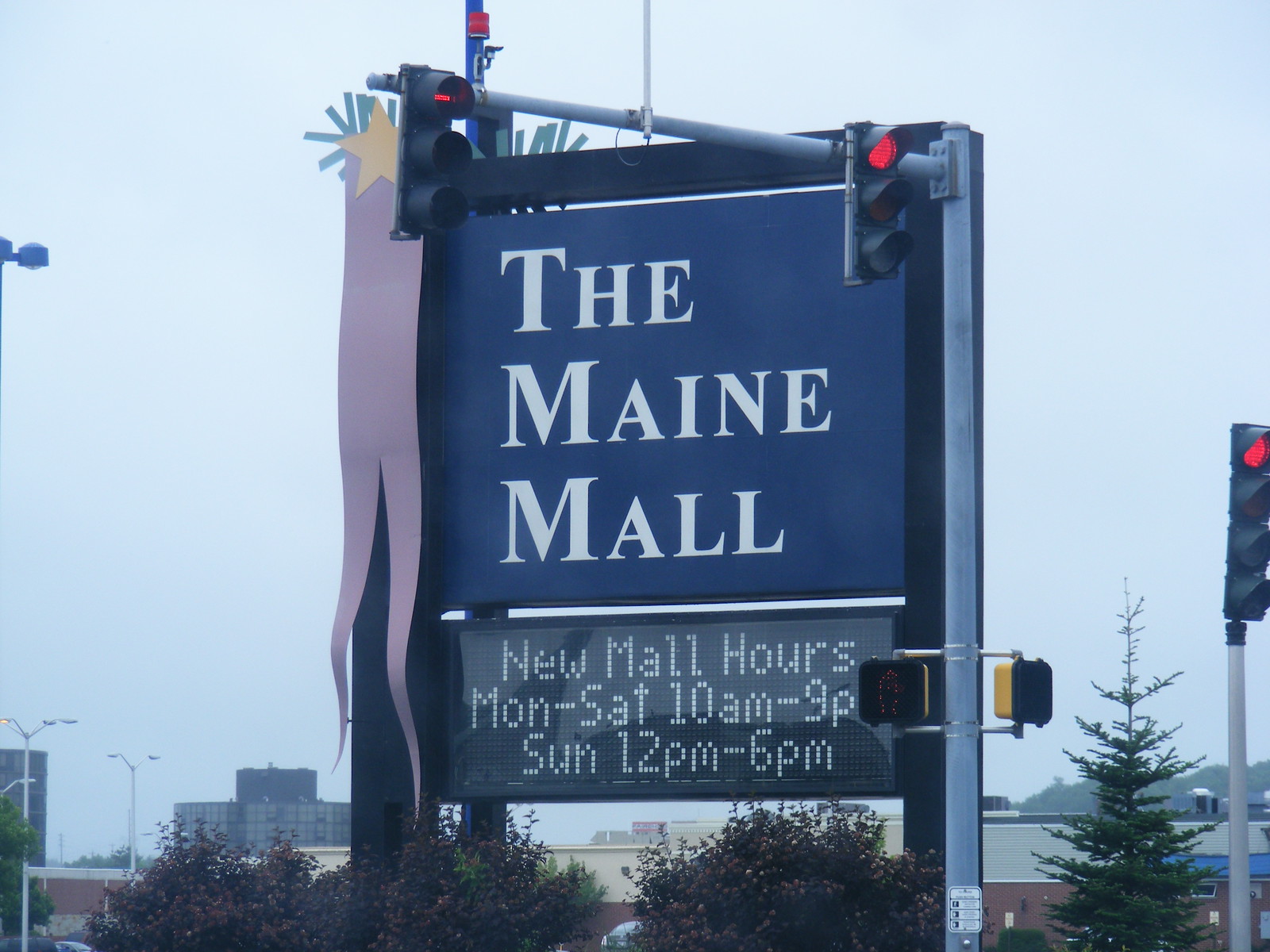A daytime photograph showcases an urban scene with exceptional image quality. Prominently featured in the center, a large, eye-catching sign stands tall. The sign has a light pink hue on one side, topped with a gold star, and features a black background with white lettering that reads "The Main Mall." Directly beneath this, a digital display provides visitors with the new mall hours: "Monday to Saturday 10 a.m. to 9 p.m., Sunday 12 p.m. to 6 p.m," in white font on a black background.

To the left, mounted on a silver metal pole, are red stoplights. Adjacent to these are the 'Don't Walk' pedestrian crossing signals. The scene is complemented by a green tree positioned towards one side of the image. Below the sign, additional red stoplights and light poles can be seen against a backdrop of industrial buildings, adding depth and context to the photograph.